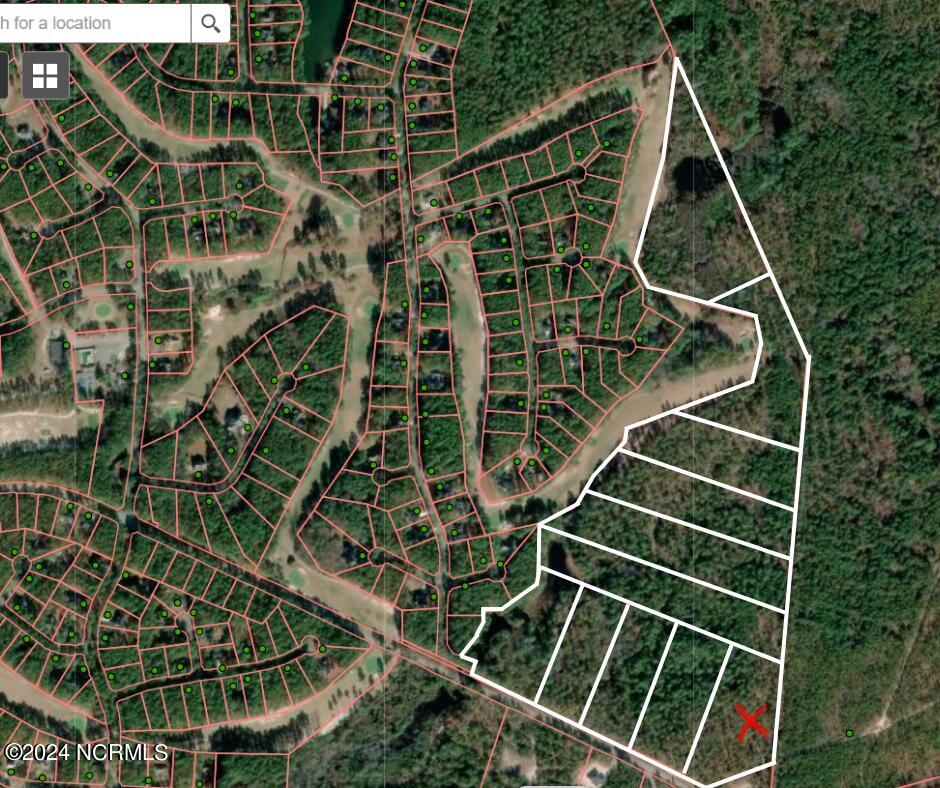The image is a top-down view of a satellite-style map reminiscent of Google Maps. The landscape is predominantly green, with a grid-like pattern overlaid, depicting various property plots. The existing plots on the left-hand side are outlined in an orangey-brown border, indicating developed areas with visible roads and fields among the greenery. Towards the right-hand side, larger plots are outlined in bold white borders, with one plot in the bottom right corner marked by a red X, seemingly drawn in Photoshop. In the top left corner, partially cut off, there is a search bar with a magnifying glass next to it, suggesting a search function, and below it is a gray icon featuring a 2x2 grid of white squares. The bottom left corner contains a copyright notice in white text, stating "© 2024 NCRMLS."